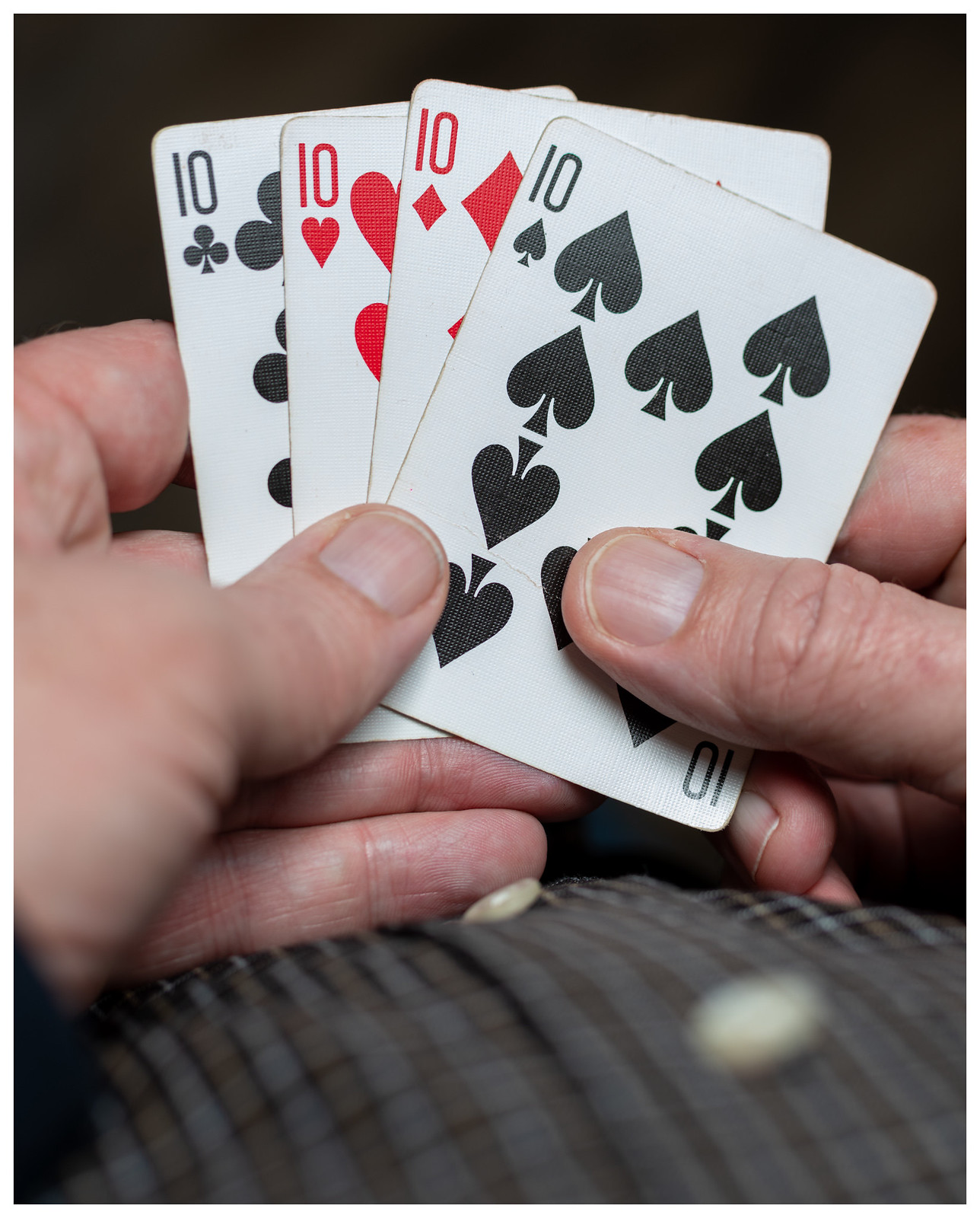A close-up photograph captures a person seated, wearing a plaid button-down shirt adorned with tight, checkered patterns in shades of brown, white, yellow, and hints of blue. The lighting fades into darkness towards the top and background of the image, adding a subtle dramatic effect. The shirt's ivory buttons are faintly visible, though the image is slightly blurred. The person's left hand is prominently featured, holding four playing cards. With their pinky, index, ring, and middle finger supporting the cards from the back, while both thumbs hold the front. The cards are fanned out to display their faces clearly: a 10 of clubs, 10 of hearts, 10 of diamonds, and a 10 of spades, evenly split between red and black suits.